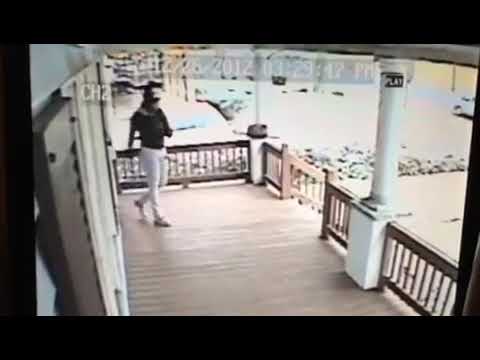The image is a still shot from a surveillance camera, framed as a wide rectangular picture with black borders on the top, bottom, and left sides. It captures an overhead view of a large front porch of a house, constructed from light brown, thin wooden slabs and surrounded by a matching brown wooden railing. On the leftmost part of the image, there are dark brown shutters on white window panes, and white pillars are visible, supporting a roof above the porch.

Positioned slightly left-of-center in the top portion of the image, a man wearing a hat, long-sleeved black shirt, and white pants is walking from left to right, appearing to head towards a staircase that descends to a pathway on the right side of the porch. The setting suggests an outdoor daytime scene in winter, reflected in the neutral tones of white, brown, beige, black, gray, and green.

At the top of the image, there is a white text overlay that reads "12-26-2012 3:29:47 PM CHANNEL 2," confirming it as a surveillance still shot taken in the afternoon on the day after Christmas, 2012.